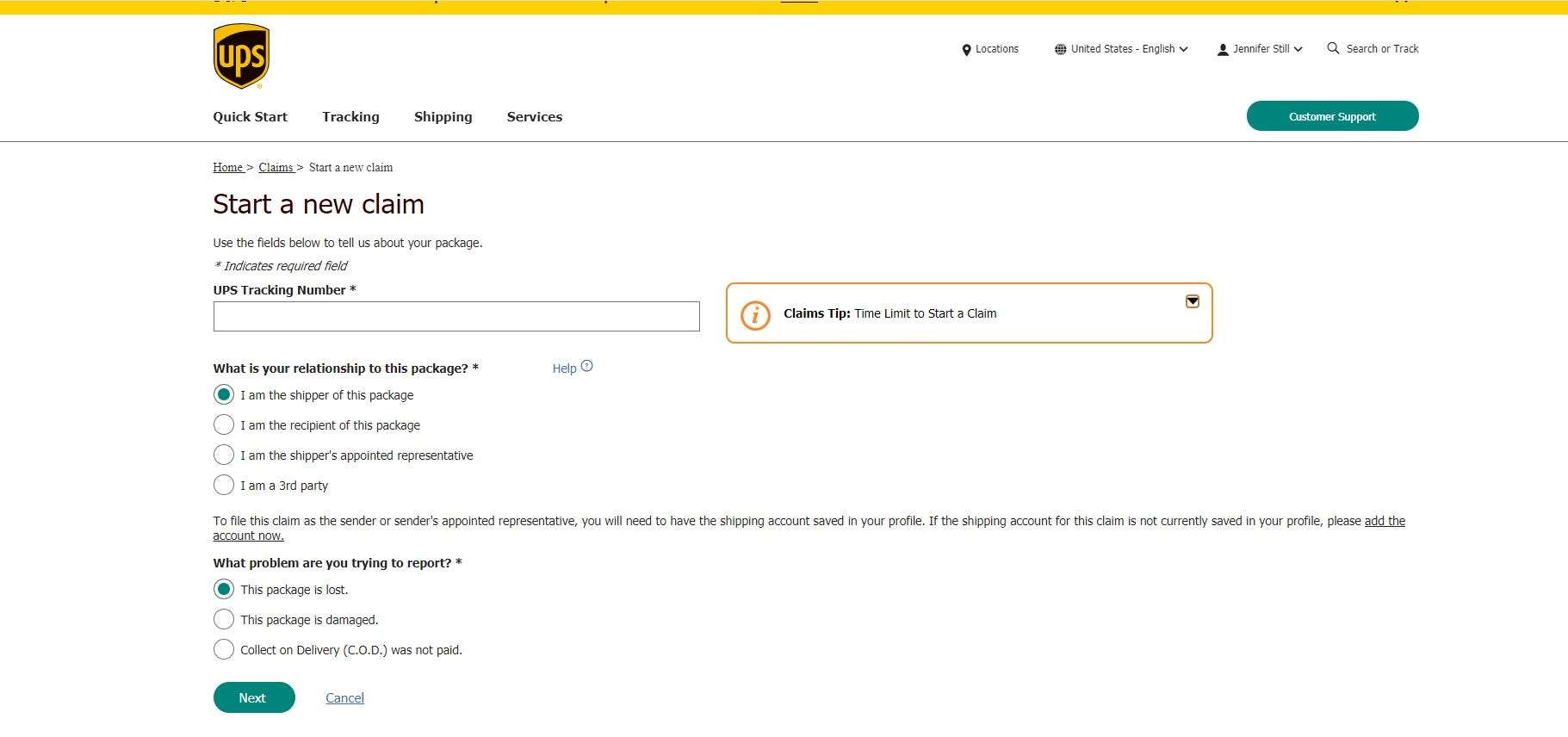The screenshot displays a UPS webpage dedicated to initiating a claim. In the upper left corner, the well-recognized UPS logo is prominently featured. Below the logo, a series of navigational tabs are presented: Quick Start, Tracking, Shipping, and Services. Below these tabs, there's a breadcrumb trail indicating the user's current navigation path: Home, followed by an arrow pointing to Claims, and then another arrow leading to Start a New Claim. 

The header of the page, in larger text, prominently reads "Start a New Claim." Instructions beneath the header prompt users to "Use the fields below to tell us about your package."

Central to the page is a blank input box where users are to enter their UPS tracking number. Adjacent to this input box, a bordered yellow box stands out with the text: "Claims Tip: Time Limit to Start a Claim."

On the left side of the page, bold text inquires, "What is your relationship to this package?" Below this are four options, each accompanied by a selectable circle. The first option, with the circle filled in, is "I am the shipper of this package." The other options, with unfilled circles, include:
- I am the recipient of this package
- I am the shipper's appointed representative
- I am a third party

Further instructions in bold warn: "To file this claim as the sender or sender's appointed representative, you will need to have the shipping account saved in your profile. If the shipping account for this claim is not currently saved in your profile, please," followed by a link labeled "add the account now."

Below these instructions, another section in bold asks, "What problem are you trying to report?" followed by an asterisk. Users are presented with three options, each with a selectable circle. The option selected by default (filled in circle) states, "This package is lost." The other two options—"This package is damaged" and "Collect on delivery (COD) was not paid"—have unfilled circles.

At the bottom of the page, two actionable buttons are displayed: a button labeled "Next" and a link labeled "Cancel."